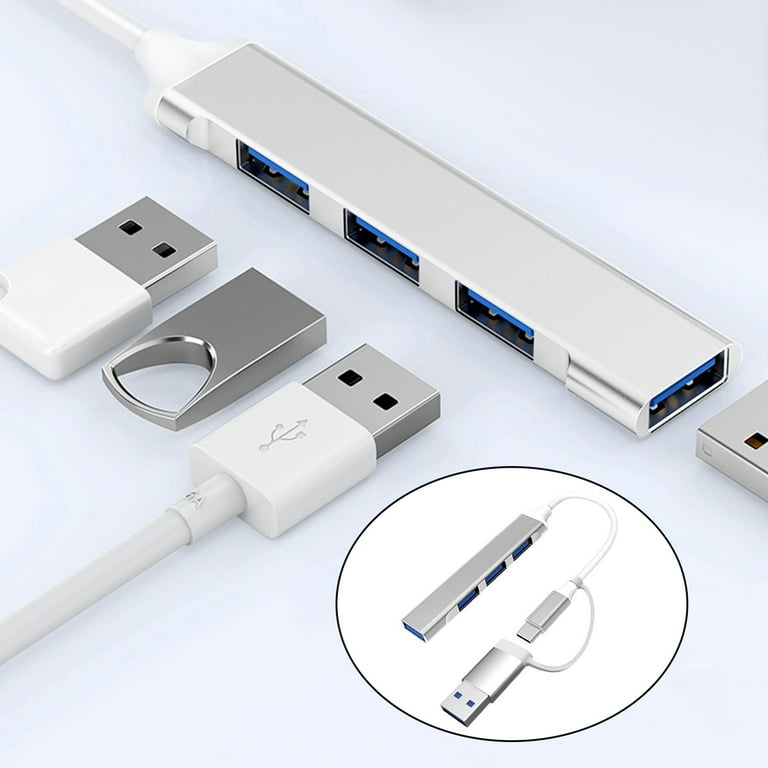The image displays a collection of USB cords and a multi-slot USB adapter, photographed from an angled, top-down perspective. The primary focus is the USB connections and a three- to four-slot USB adapter dock, prominently situated at the top of the light gray background. The adapter features one slot on its right side, three on the left, and one at the end. In front of the adapter are three different USB devices: a white USB plug with a silver, shiny connector, positioned diagonally up and to the right; a small, silver metal USB key to its left; and a white USB thumb drive. Highlighting one of these USB cords is a distinct black ring encircling a white circle. The image includes a variety of colors such as blue, black, white, silver, gray, and off-white, and it's not clear whether it was taken indoors or outdoors, or even digitally created.